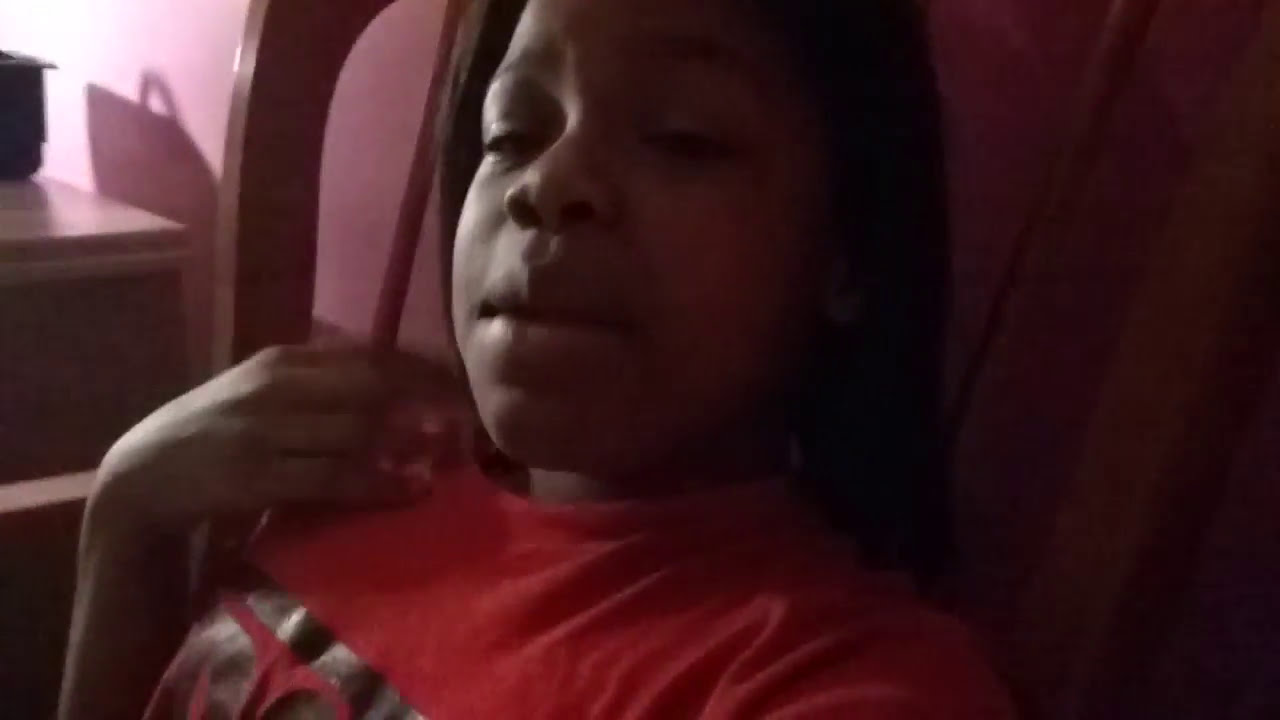The image depicts a young black woman with smooth, dark skin sitting indoors in a wooden chair, visible only from the shoulders up. She is situated in the center of a wide, rectangular frame. Her head is slightly turned to the left with partially open eyes and her mouth somewhat ajar, giving her a tired appearance. She has large lips, thin black eyebrows, and long black hair cascading down her back. The woman is wearing a red t-shirt with a partially visible black design towards the bottom left corner of the image, and her left hand is raised, touching her shoulder. The chair features a thick wooden backrest with horizontal wooden poles. Behind her is a reddish-pale wall. On the left side of the image, a light brown wooden dresser is visible, topped with what appears to be a black electronic object casting a shadow to its right. The image suffers from low quality and low-light conditions, with soft focus and noticeable compression artifacts, indicating it might have been taken with a struggling camera, potentially as a selfie. The color palette includes shades of red, brown, black, and gray.